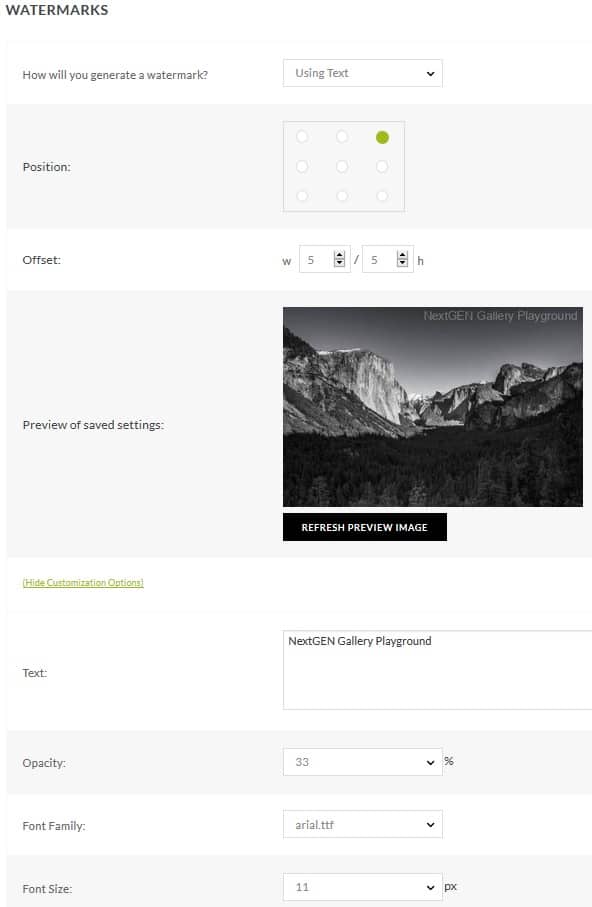This screenshot, likely from a website interface, primarily features an all-white background with sections distinguished by light gray boxes. At the top, there's a header titled "WATERMARKS" in bold, black, uppercase letters. Directly below this, a question is posed in black text: "How will you generate a watermark?"

Following the question, a gray-outlined box contains the text "Using text" inside it, pointing downward with an arrow. Beneath this, another light gray box on the right side includes the word "Position" in black font. Within this section, a large off-square grid with nine white circles, each outlined in gray, is displayed. One of these circles is solid green, indicating a selected position.

Further down, the interface includes an "Offset" section providing various measurement options. Below this section, there is another gray-outlined box displaying a black and white image of a mountain. At the bottom of this box, a black button labeled "Refresh Preview Image" is visible.

Underneath the preview image box, there is a clickable green text link. Finally, a set of options is presented for users to create their watermark.